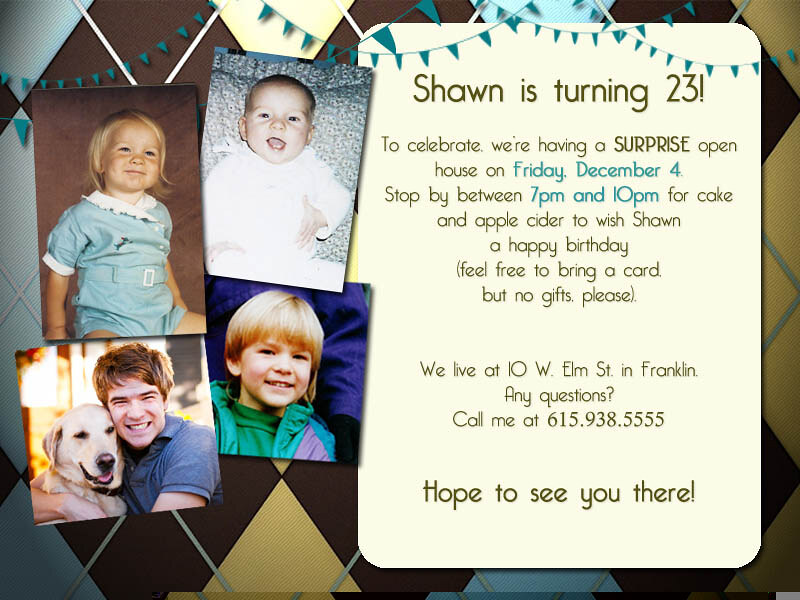The image serves as an invitation to celebrate Sean's 23rd birthday. On the left side, a series of photos show Sean's growth over the years: as a baby, a toddler, a young child around five, and finally, a young adult in his 20s smiling and hugging a Labrador Retriever. The background features a festive diamond pattern and celebratory pennant banners at the top. On the right, there’s a white text box with an invitation message that reads: "Sean is turning 23. To celebrate, we're having a surprise open house on Friday, December 4th. Stop by between 7 p.m. and 10 p.m. for cake and apple cider to wish Sean a happy birthday. Feel free to bring a card, but no gifts, please. We live at 10 West Elm Street in Franklin. Any questions, call me at 615-938-5555. Hope to see you there." The overall design resembles a postcard, making it a cheerful and inviting announcement for Sean’s special day.